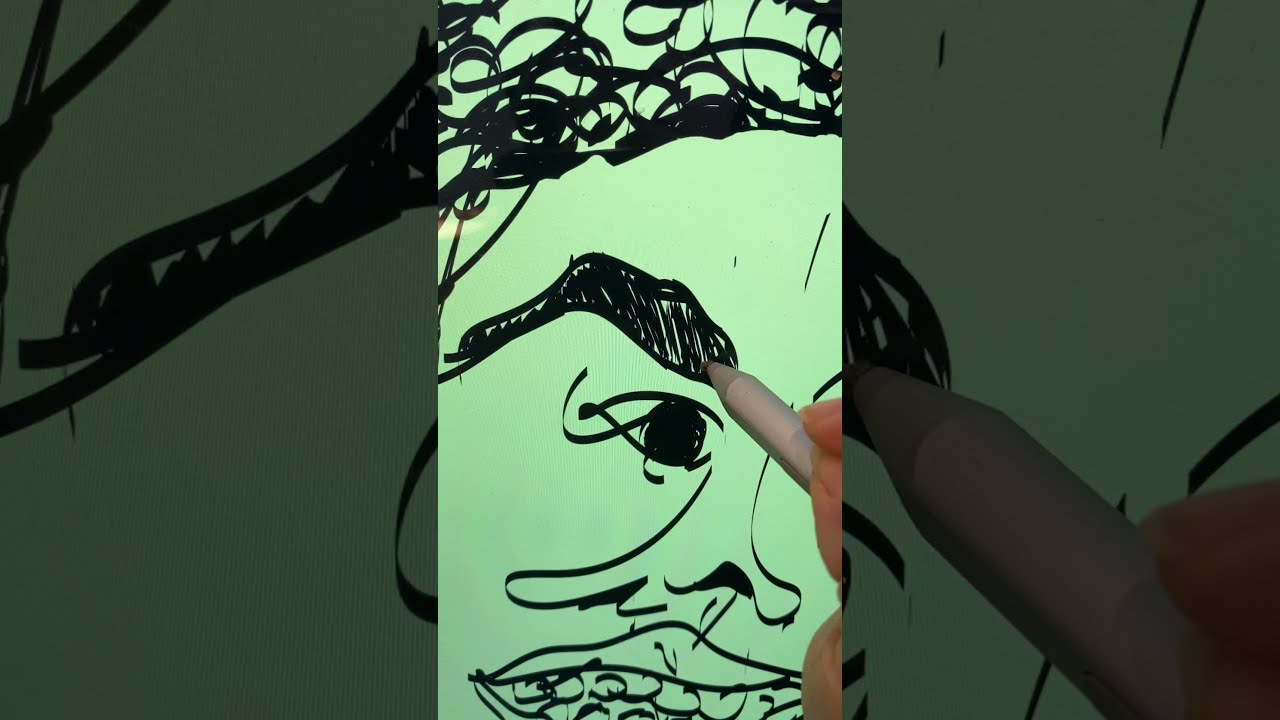The image is a detailed artwork segmented into three vertical sections. The central section showcases a sketch or painting of a face created with black ink or marker on a light green background. This visage features distinct, unconventional shapes for facial features: thick black curly hair, a prominent eyebrow that is being actively sketched by a light purple pen held in a pair of Caucasian fingers, eyes, a sloped nose, and a peculiar mouth with exaggerated circular teeth and a single, undefined upper lip. The left and right sections of the image are enlarged, darker close-ups of the respective sides of the central portrait. The color palette is limited to green, black, gray, and tan, contributing to the unique aesthetic of the artwork. The image does not contain any text and appears to be a digital or scanned piece of art, possibly captured from a mobile device.